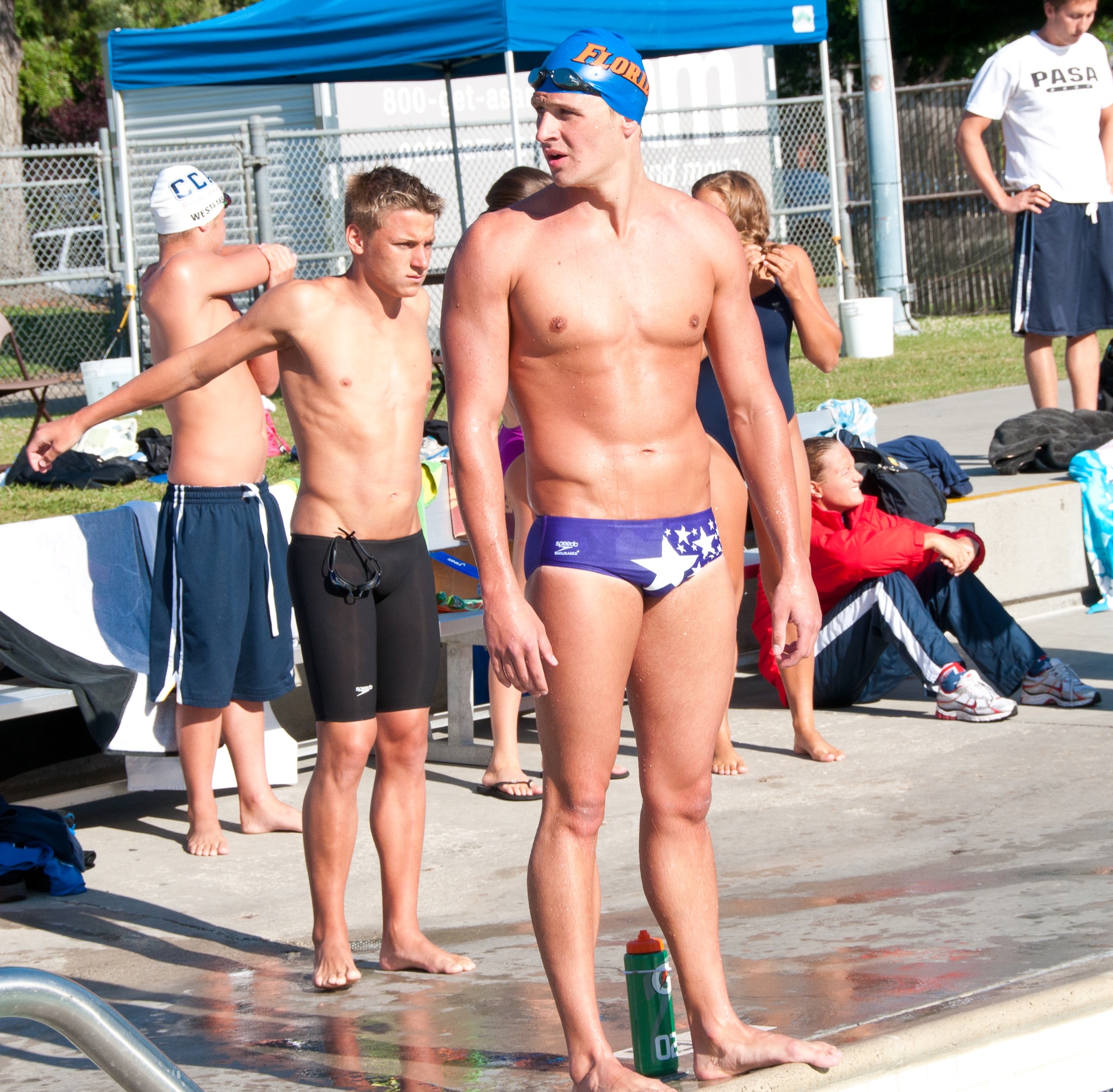The image captures the intense prelude to a competitive swimming race. At the edge of the pool stands a muscular young man, clad in blue swim trunks adorned with white stars and a matching blue skull cap that reads "Florida" in orange letters. His swimmer's goggles rest on his head as he gazes to his left, poised and ready. Behind him, a shorter athlete stretches, wearing longer blue swim trunks with his goggles looped around his waist. The poolside is bustling with athletes and spectators; the wet, darker patches on the ground hint at recent activity. In the backdrop, a chain-link fence and a blue pop-up canopy frame the scene, under which a person in a white shirt emblazoned with "PASA" and black shorts stands hands-on-hips, overseeing the preparations. The field of grass beyond features more swimmers gearing up, their white caps marked with "C-C" as they stretch and ready themselves. Prominent in the foreground is another swimmer in purple tights with white stars, a blue cap with "Florida" in yellow, and goggles perched on his head, emphasizing the communal and competitive spirit of the event.